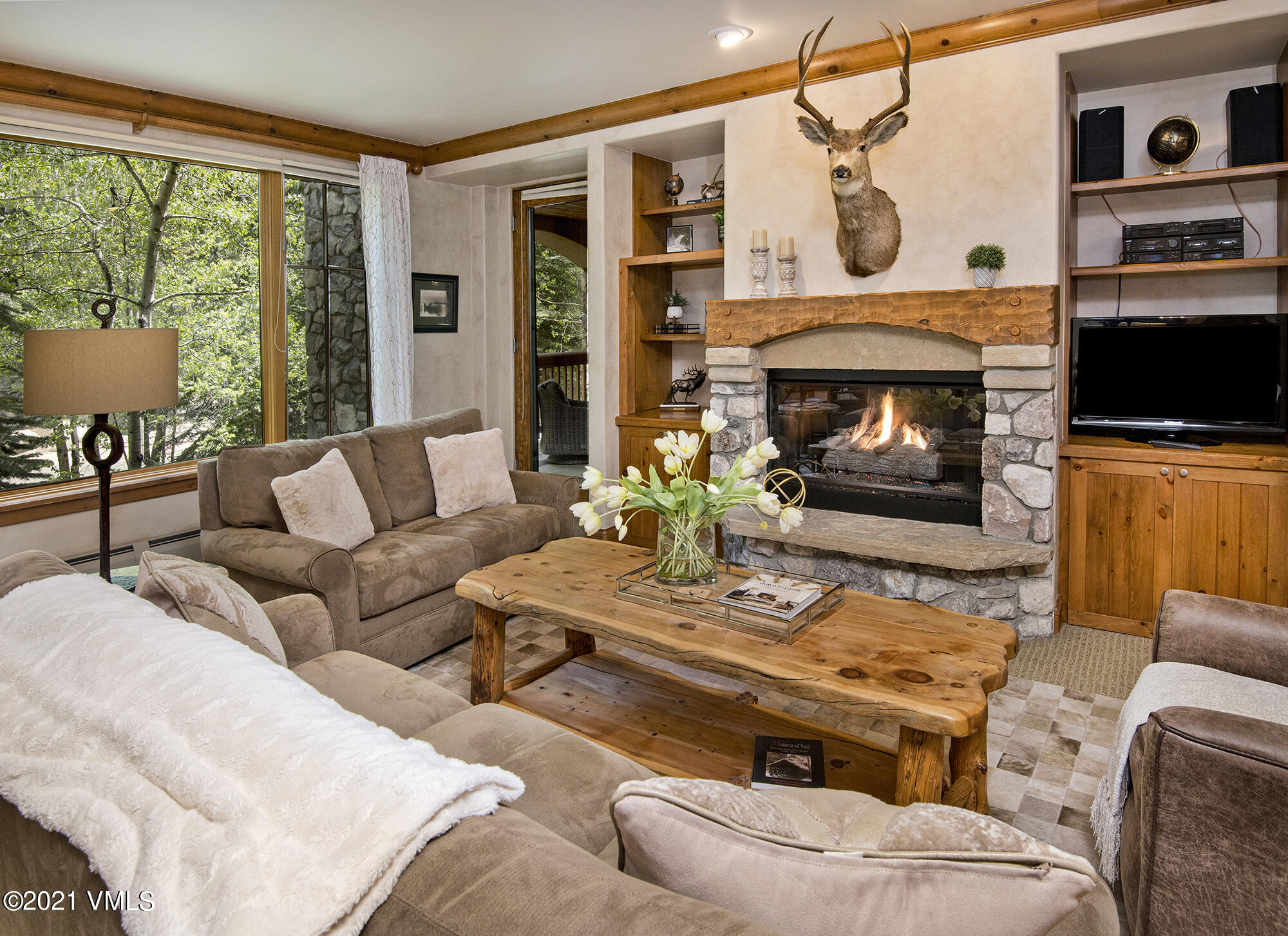This detailed photograph captures a cozy, rustic indoor living room, likely within a cabin nestled in the forest. The central focus is a wooden coffee table adorned with a vase of white tulips and some magazines. Behind it stands a lit stone fireplace with a wooden mantle, above which hangs a prominent deer head with antlers. Flanking the fireplace are recessed wooden shelves; the left shelf is filled with decorative knickknacks and statues, some resembling deer, while the right shelf houses a small TV set, speakers, and electronic equipment. A golden atlas sits between the speakers on a higher shelf. 

To the right of the fireplace, a comfortable leather chair is visible near the table. On the left side of the room, a large picture window offers views of dense, verdant trees outside, enhancing the cabin’s secluded ambiance. In front of and to the left of the coffee table, you can find additional seating including a long beige couch complemented with a white afghan and pillows, and a light brown loveseat. The beige walls and wood accents throughout the room further contribute to the warm, inviting atmosphere. An off-white rug covers part of the tan floor, adding to the room's rustic yet cozy charm.